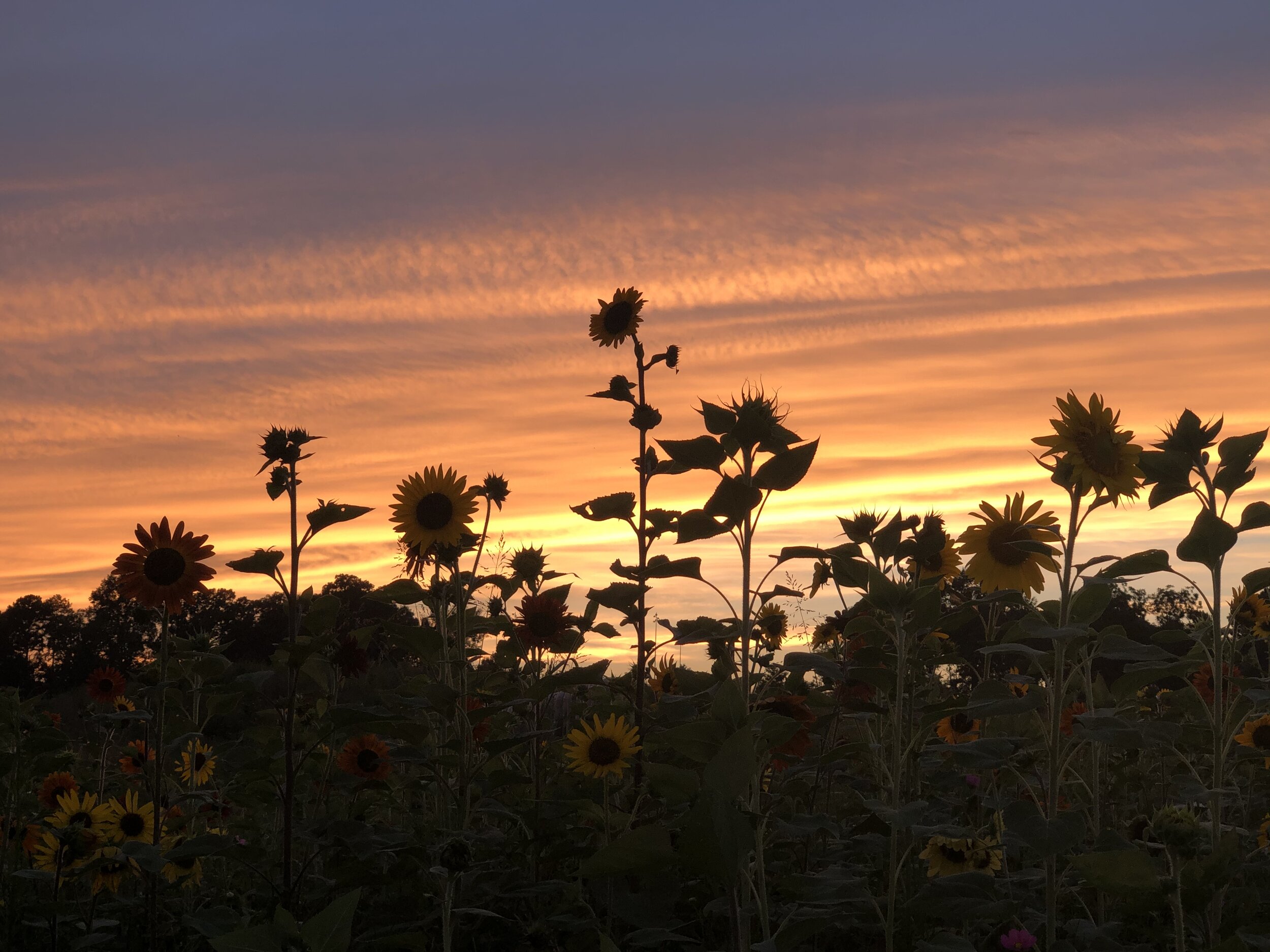This photograph captures a stunning scene at either sunrise or sunset, featuring a vibrant display of colors in the sky. Starting from the horizon, the sky transitions from streaks of bright yellow to deep orange, and finally to a purplish-blue at the top. In the foreground, a field of sunflowers stretches across the frame, their dark silhouettes contrasting against the luminous background. Most of the sunflowers are in full bloom, with visible stems and leaves adding texture to the scene. One particularly tall sunflower stands prominently in the middle, drawing the viewer's focus. Although the sunflowers appear dark due to the intense backlighting, you can faintly discern their yellow petals. The sky is streaked with clouds that are arranged in slightly askew rows, adding to the artistic composition of the image. A small, indistinguishable building is barely visible on the right side of the frame, blending into the darker parts of the photograph. The image overall strikes a delicate balance between shadow and light, capturing the serene beauty of the natural world.